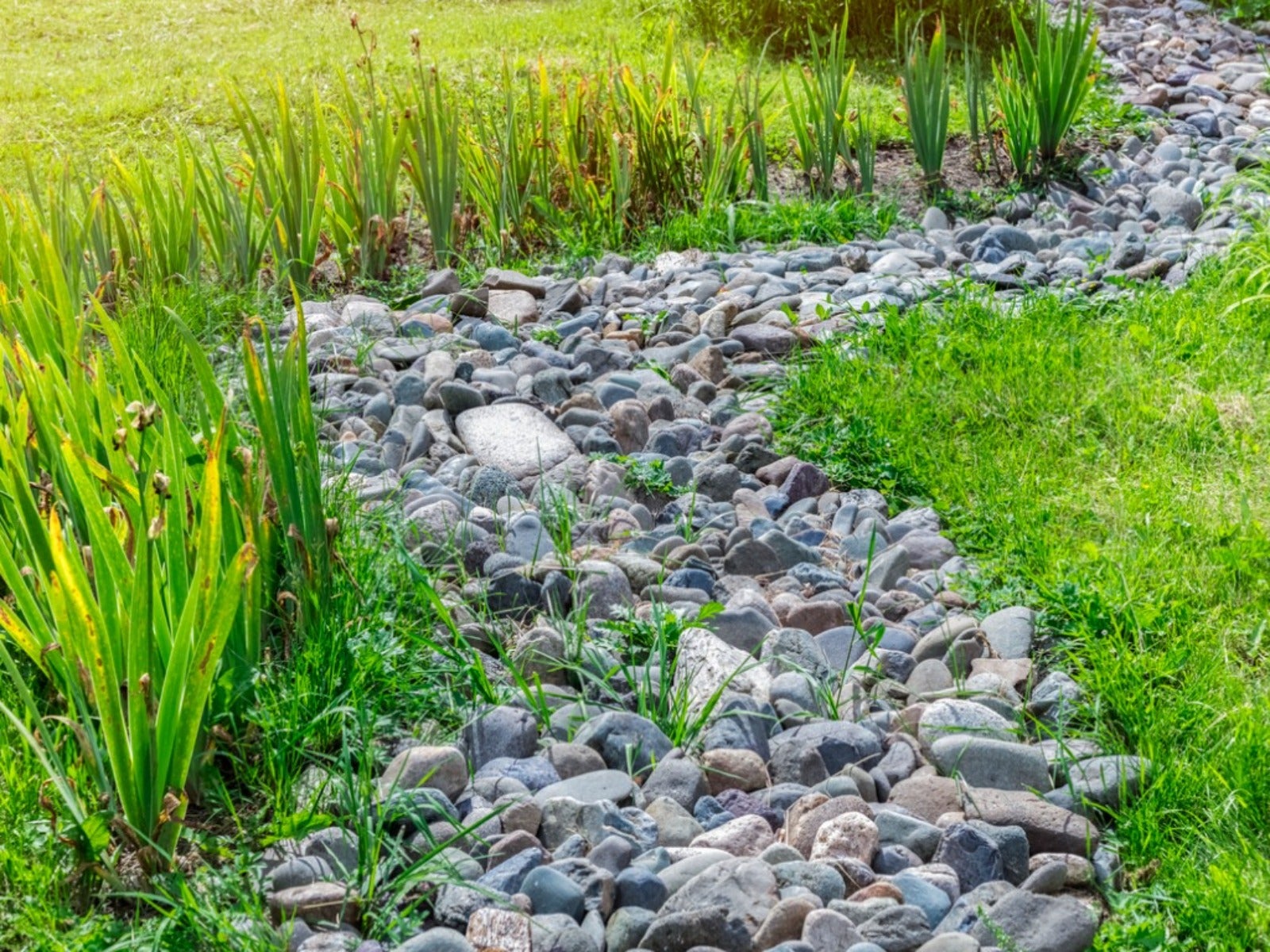This outdoor photograph is captured in a landscape layout, showcasing a winding stone pathway that notably mimics the serpentine curves of a snake. The pathway, composed of an assortment of rocks and large boulders ranging from two to six inches in size, primarily features hues of dark gray, beige, white, and occasional blues. The stones present a variety of textures: smooth, rough, and even some with holes. The path initiates at the bottom of the image, veers slightly right, then takes a subtle left turn before curving back to the right, eventually leading the viewer's eye to the upper right-hand corner of the photo.

The left side of the pathway is bordered by tall grasses and cattails, which create a natural barrier and, beyond them, there extends a lush green field. On the right side, the rocky path is flanked by wild grass. Scattered intermittently, small blades of grass and weeds peek through the gaps between the stones, adding to the organic, untamed feel of the scene. The simplicity of the composition is unobstructed by human presence or additional elements, allowing the natural colors of the rocks and the vibrant green of the grass to dominate the image.